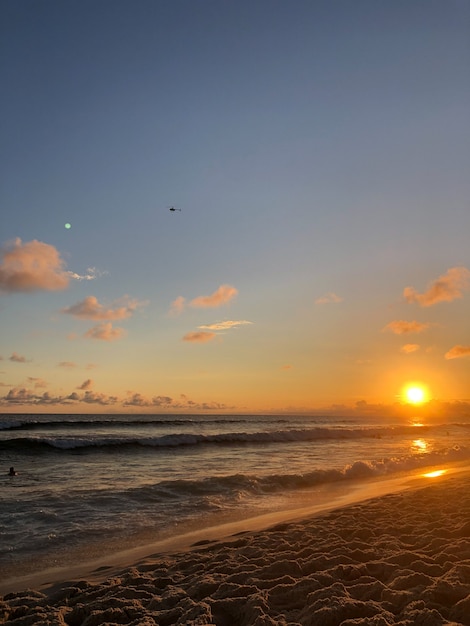This is a detailed image, possibly a photograph or a painting, depicting a beach scene during sunset or sunrise. The captivating scene features an orange sun positioned just above the horizon on the right side, casting a striking yellow and orange glow across the sky. Encircling the sun, the sky transitions from a bright yellow to a lighter blue, gradually darkening to a deep blue at the top. Subtle clouds pepper the lower half of the sky, and a faint silhouette of a small helicopter hovers slightly left of center, adding an element of intrigue.

Below the horizon, the choppy ocean waves reflect the colorful sky as they approach a dark, well-trodden sandy beach adorned with divots and ripples. Small, frothy whitecaps are visible on the waves, which suggest a sea or ocean rather than a lake. In the distance to the left, a moon or another celestial body is barely visible, enhancing the image's moody and serene atmosphere. There appears to be a silhouette of a person or object, possibly a buoy, in the water on the left side. The overall hue of the image is dark and moody, capturing the transitional beauty of twilight over an active beach scene.